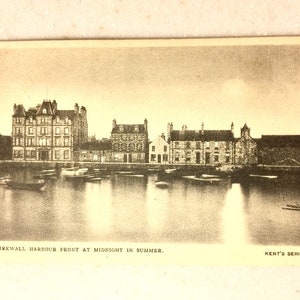The image is a photograph of an old, yellowed postcard or photograph set against an off-white surface. The black and white image captures a waterfront scene, likely taken during the daytime, featuring a body of water with numerous small boats and dinghies either docked or floating. Across the water, a series of Victorian-style buildings are visible. On the far left, a large, possibly four or five-story building with multiple rows of windows stands prominently. Adjacent to it on the right is a smaller, less detailed structure, followed by three more buildings of average height, with the central one being slightly shorter than the others. In the distance behind the buildings, there are trees, and the sky appears hazy or smoggy. The bottom of the photograph features a partially cut-off caption that hints at "Blank Harbor Front at Midnight in Summer," with the word "Kent" partially visible before being cut off. The detail and composition suggest this image captures a nostalgic, serene waterfront, frozen in time.